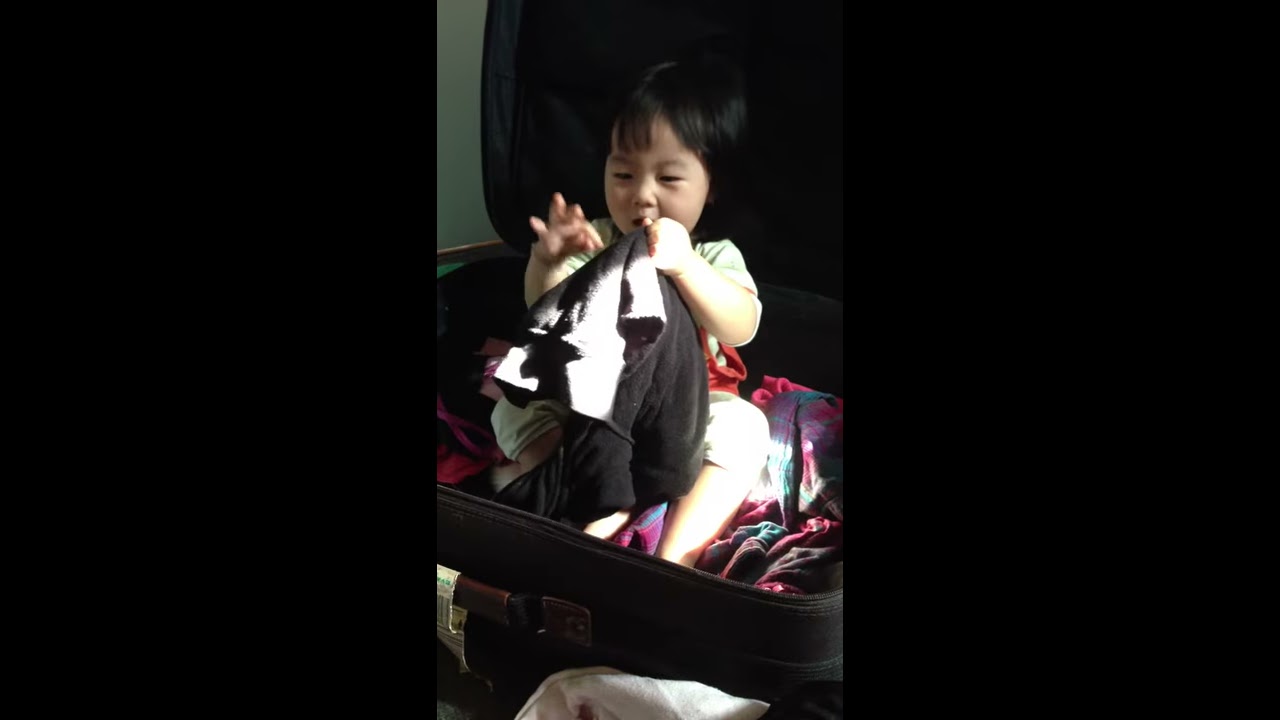This photograph centers on a young Asian girl, possibly of Chinese descent, who appears no older than two years. She is seated inside an open black or dark gray suitcase, surrounded by and sitting on various colorful pieces of clothing. The child, with her short black hair and clad in a light-colored top and shorts, is positioned directly in the center of the suitcase, which takes up most of the image. She holds up a dark gray or black sweater close to her lips, seemingly sucking on it. The suitcase, only partially filled, displays its brown handle at the lower part of the image. The scene, most likely set indoors in a bedroom or closet during the day, has no other significant objects or text, emphasizing the playful and innocent moment captured.